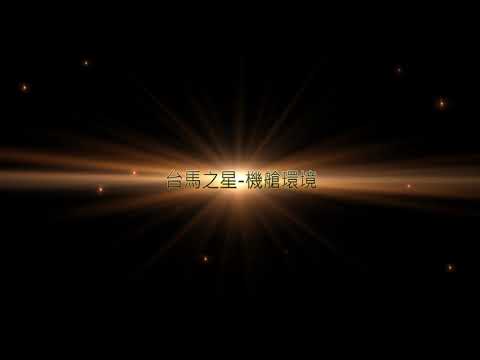The image depicts an ethereal, space-like scene, dominated by a simple black background that evokes the depths of outer space. Central to the image is a luminous golden starburst, radiating light in all directions with a brighter concentration in the middle, which fades as it extends outward. Embedded within this radiant starburst are Chinese or possibly Japanese characters, prominently outlined in black that contrasts sharply against the glowing light. Accentuating the celestial theme, scattered across the scene are smaller golden and white stars, some faint and distant, others more prominent, contributing to the tranquil and otherworldly atmosphere of the image. This composition resembles a cinematic opening scene, capturing the viewer's attention with its radiant beauty and cosmic allure.